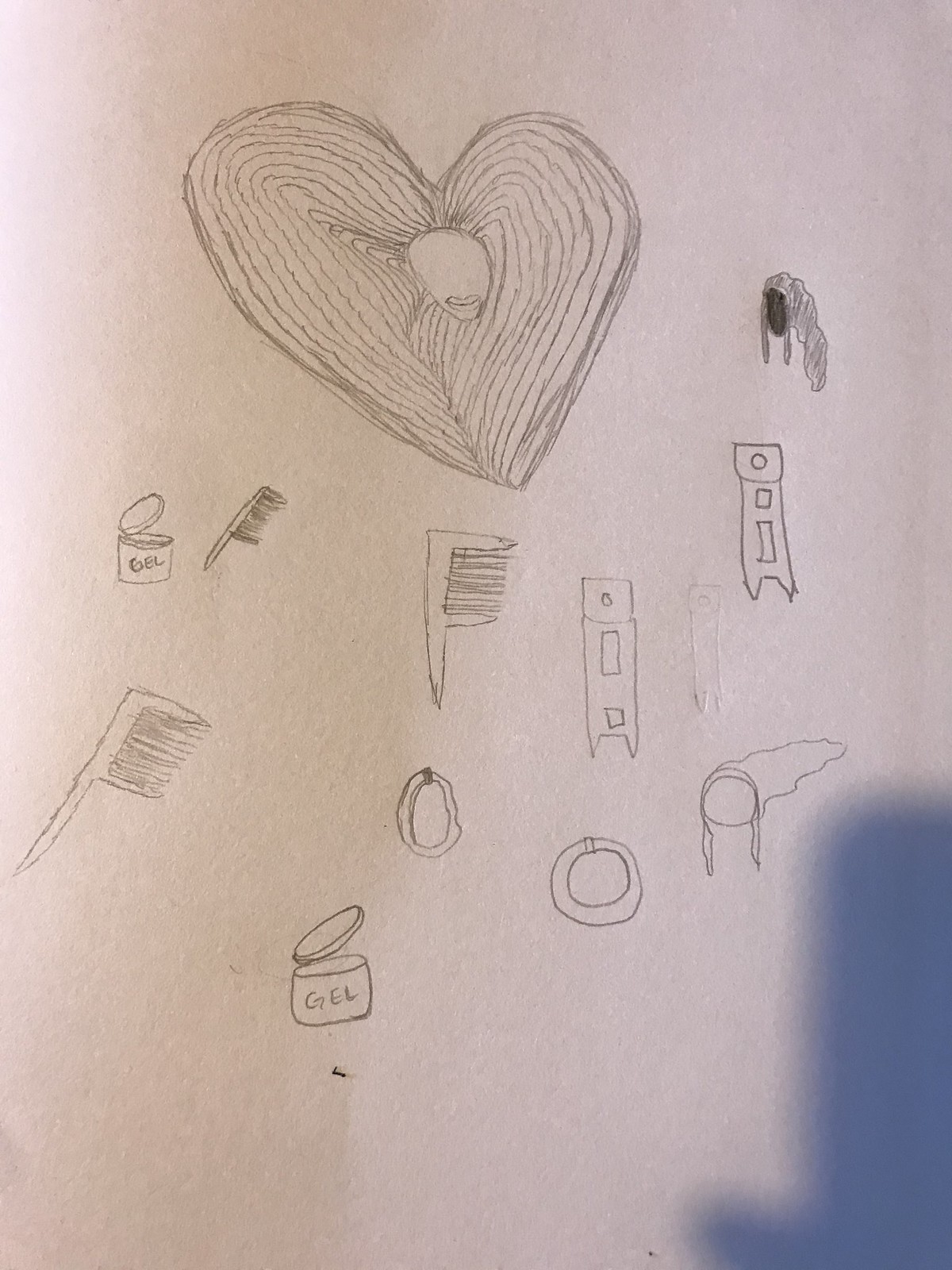The image displays a series of black-lined drawings on a gray piece of paper. At the bottom, there's an open container labeled "gel." Above it and to the right, two rings are depicted. Further to the right, a cloud is illustrated with strings extending from both sides. On the left side of the image, there is a diagonal comb with its teeth pointing right, and another similar comb situated above it. Another open gel container is positioned further above to the left. To the right, the image includes shapes comprising a square, rectangle, and circle. Above these shapes, a black-shaded oval is seen, with a cluster of gray shading adjacent to it. Additionally, a heart with dark gray lines running through it is situated to the left of the oval. The paper has a dark blue shadow in the bottom right corner, adding depth to the overall composition.